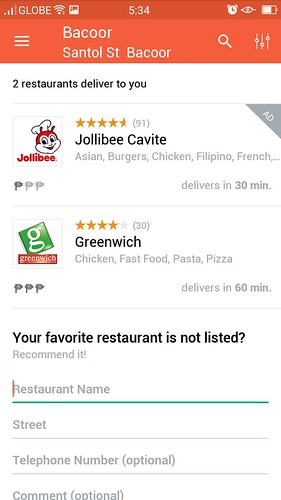This descriptive caption details a smartphone screenshot with an orange and light orange border. At the top of the screen, there are icons for Wi-Fi, battery, a globe, and a picture. Additionally, there are icons for a timestamp of 5:34, an alarm icon, an eye-shaped icon, and another battery indicator. 

In the lighter section at the bottom, on the left, there is a hamburger icon. To the right of the hamburger icon, the text reads "Bacore, St. Bacore," followed by a search icon, and three lines with circles that symbolize a slider for options. 

In the main body of the screenshot, which has a white background, there is text stating "Two restaurants delivered to you."

1. The first restaurant listed is Jollibee, represented by a logo of a bee wearing a chef's hat. It boasts a rating of 4.5 stars out of 5 based on 91 reviews and offers Asian burgers, chicken, Filipino cuisine, and French dishes, promising delivery within 30 minutes.

2. The second restaurant listed is Greenwich, identified by a logo featuring a green box with a white "G" and a red banner beneath it with the text "Greenwich." It has a rating of 4 stars out of 5 from 30 reviews and provides chicken, fast food, pasta, and pizza, with a delivery time of 60 minutes.

At the bottom, there is an option to search for your favorite restaurant if it is not listed.